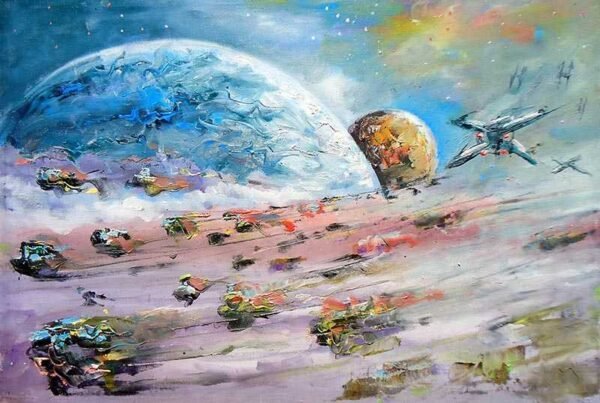This oil painting captures a vivid, futuristic sci-fi scene set on an alien planet with a distinctive purple-white hue. The view overlooks a dynamic battlefield filled with various spacecraft and ground vehicles speeding by. Among the chaos, some of the ships resemble X-wings from Star Wars, while others feature unique designs, including X-shaped fighters and blue and black motorcycle-like vehicles, many of which are airborne. The scene is bathed in a cascade of vibrant colors—reds, pinks, blues, greens, yellows, and oranges—creating a brilliant, stylized space sky. Dramatic celestial bodies dominate the background, including a close, large blue planet and a smaller, yellow one behind it. Despite the low resolution, the painting vividly depicts a scene of high-speed aerial combat and interplanetary adventure.